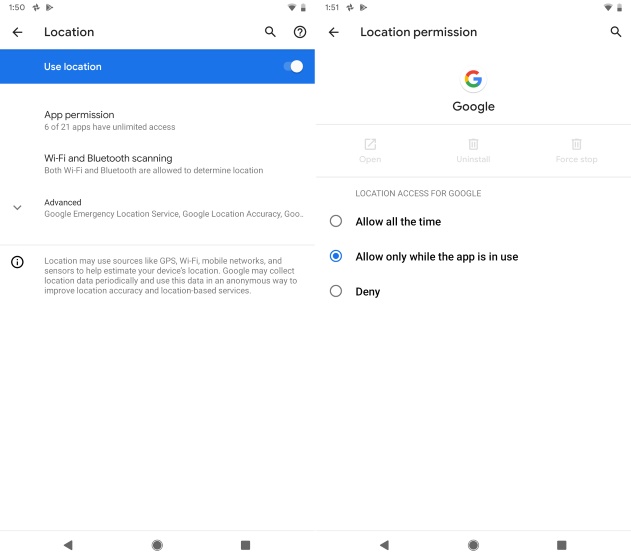The photographic image showcases a side-by-side comparison of screenshots taken from a mobile device.

**Left Screenshot:**
- **Time:** 1:50 PM, displayed in the upper left-hand corner.
- **Signal & Battery:** The Wi-Fi signal shows two bars, and the battery is at approximately 40%.
- **Navigation & Location Details:** An arrow pointing to the left is present, with "Location" written at the top in black font.
- **Iconography & Prompt:** A magnifying glass encircling a question mark appears, adjacent to a blue banner stating "Use location" with the toggle switch turned on.
- **App Permissions:** Indicates that six out of 21 apps are utilizing unlimited access to location services.
- **Wi-Fi & Bluetooth Scanning:** A section dedicated to Wi-Fi and Bluetooth scanning.
- **Advanced Options & Info:** An advanced options dropdown indicated by a downward arrow. There is also an informational button explaining how location services may employ GPS and Wi-Fi.

**Right Screenshot:**
- **Time:** 1:51 PM, displayed in the upper left-hand corner.
- **Signal & Battery:** The Wi-Fi signal and battery indicator remain the same as in the left screenshot.
- **Location Permissions:** The screen covers location permissions, containing an arrow pointing left and a Google search bar featuring the colors green, blue, yellow, and red.
- **Location Access Options for Google:** Displays options for location access for Google, including "Allow all times," "Allow only while using the app," and "Deny."

This detailed comparative view vividly illustrates the configuration and permissions related to location services on the mobile device.